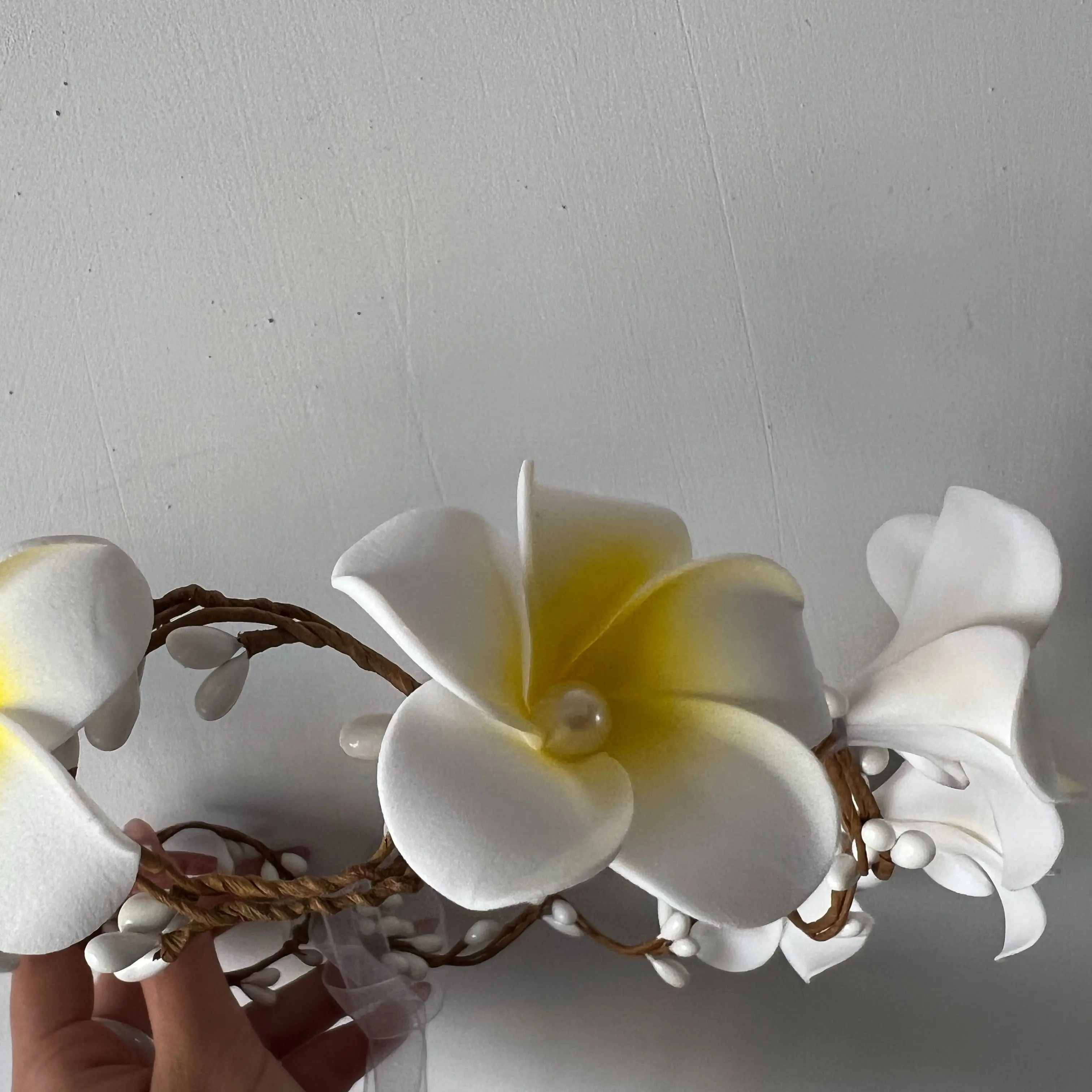In this image, a person is holding a decorative wreath in front of a stark white wall. The wreath features three to four large white blooms that resemble gardenias, creating an elegant and sophisticated look. The material of the wreath appears to be a flexible rope or another malleable substance, designed to maintain a circular shape. The white flowers, with their intricate petals, elevate the visual appeal of this ornamental piece. The background wall's simplicity accentuates the detailed craftsmanship of the wreath, making the flowers stand out prominently. The overall composition suggests a poised and stylish decor item, perfect for enhancing an interior space with its delicate charm.